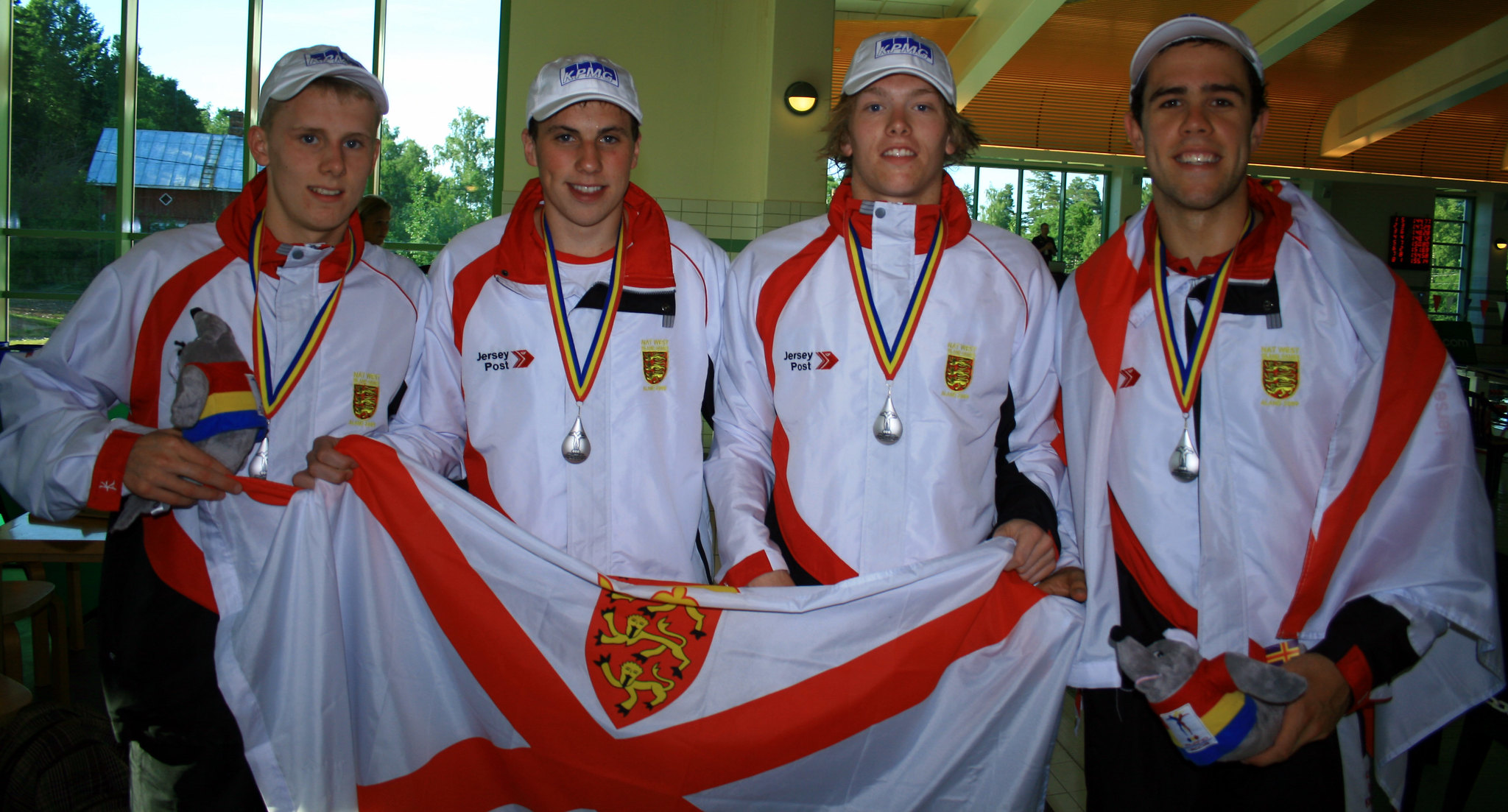This color photograph, taken in landscape orientation, captures four young men, likely high school boys, who appear to be an athletic team. They are all dressed in matching white uniforms with long sleeves, red collars, and a distinctive red stripe down the chest. Each uniform features an emblem on the left chest and the name "Jersey Post" on the right chest. The boys are all wearing award ribbons around their neck, each adorned with a silver medallion. 

Three of the boys on the left hold a white flag draped in front of them, which showcases a red X banner. At the top of the X is a red shield adorned with yellow lions, signifying a likely British emblem. The boy on the right drapes a similar flag over his shoulders. Additionally, a couple of them hold stuffed toys resembling squirrels or chipmunks, perhaps as mascots or trophies. 

Behind them, the setting transitions from indoors to outdoors, with an array of buildings and trees visible in the background. The boys are looking up at the camera, smiling, possibly celebrating a victory shortly after an award ceremony. The photograph exemplifies representational realism, capturing the moment in vivid detail.